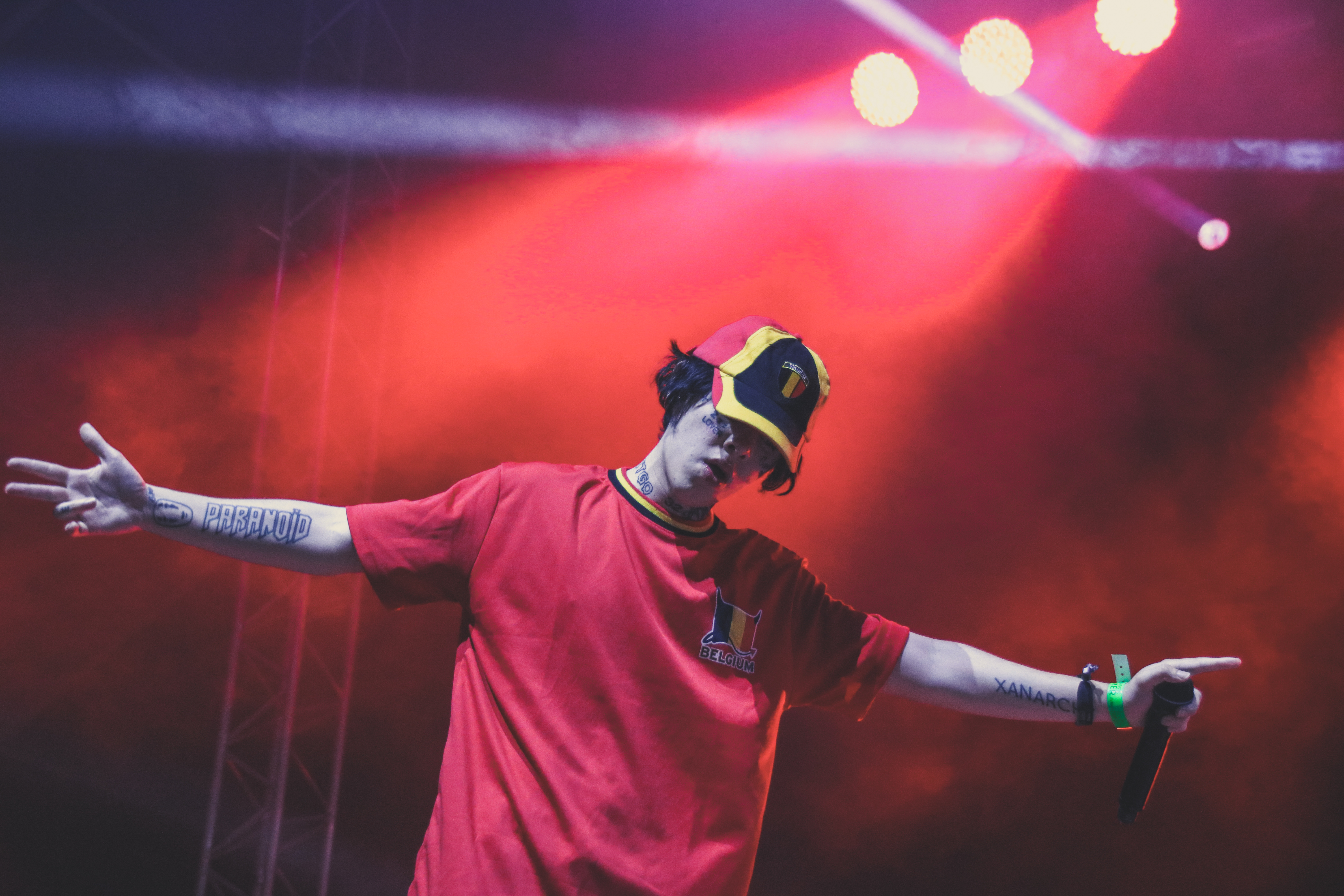The image captures the electrifying atmosphere of an indoor concert, bathed in red lighting and a misty ambiance that adds an air of mystique. Stage lights shine dramatically down, illuminating the performer beneath a horizontal white light that slices across the upper part of the scene. Dominating the foreground, a rapper stands with arms spread wide, head slightly bowed. He sports a distinctive red baseball cap with a black front panel and a yellow border around the bill and crown, complementing his vibrant red t-shirt. The t-shirt features black and yellow bands around the neck, suggesting a sports theme with a square-shaped logo on the front that includes the Belgian flag and the word "Belgium." His left hand clutches a microphone, adorned with a green wristband and another bracelet. His forearms are inked with tattoos – "paranoid" on the right and "anarchy" on the left. Additional tattoos decorate his neck and beneath his right eye. The steel girder-like beam to the left of the stage reinforces the industrial vibe of the setting, completing the dynamic portrayal of this captivating concert moment.